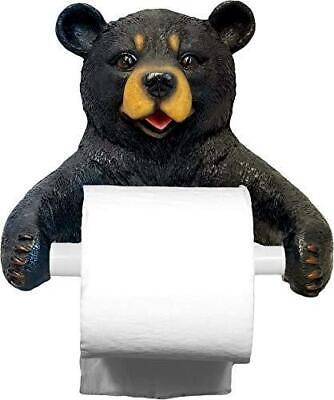This image features a charming black bear toilet paper holder designed for novelty decor, perfect for adding a playful touch to your bathroom. The black bear, with its cute circular ears and nearly smiling expression, has a distinctive light brown nose and matching light brown accents above its expressive dark brown eyes. Notably, the bear's tongue, half-sticking out, adds a whimsical touch with its pinkish-red hue, while the slightly copper-colored claws add a subtle contrast to the predominantly black body. The bear's outstretched arms hold a white, presumably plastic pole between its paws, designed to hold a roll of toilet paper. The toilet paper roll is full and positioned so that it unfurls from behind, making it easy to pull down. The bear itself appears to be made of plastic with a shiny, textured finish, especially noticeable on its head, adding a sense of detailed craftsmanship to the piece. Set against a completely white background, this humorous and practical toilet paper holder is ideal for a product listing on sites like Amazon or eBay.